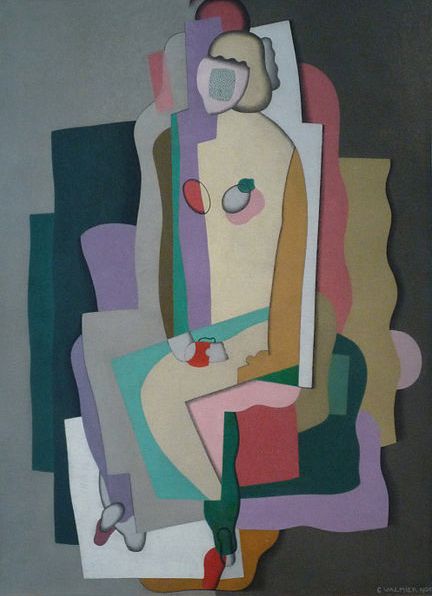This image is a detailed abstract piece of cubist art, reminiscent of a Picasso style, which you might find in an art gallery. It features a multicolored, geometric figure that is discernibly a person, albeit with no distinct facial features. The body is composed of various shapes and segments, giving it a layered, stacked appearance similar to cut-out pieces of construction paper. Notably, there are two oval shapes that represent the breasts, and the figure appears to be seated with hands in its lap.

The color palette is rich and varied, incorporating shades of purple, white, beige, black, yellow, red, tan, green, blue, and different shades of pink. The background further adds to the complexity with layers in white, brown, yellow, purple, light gray on the left, and dark gray on the right. The entire composition is very boxy and segmented, enhancing the constructed, paper-like aesthetic of this very detailed and textured artwork.